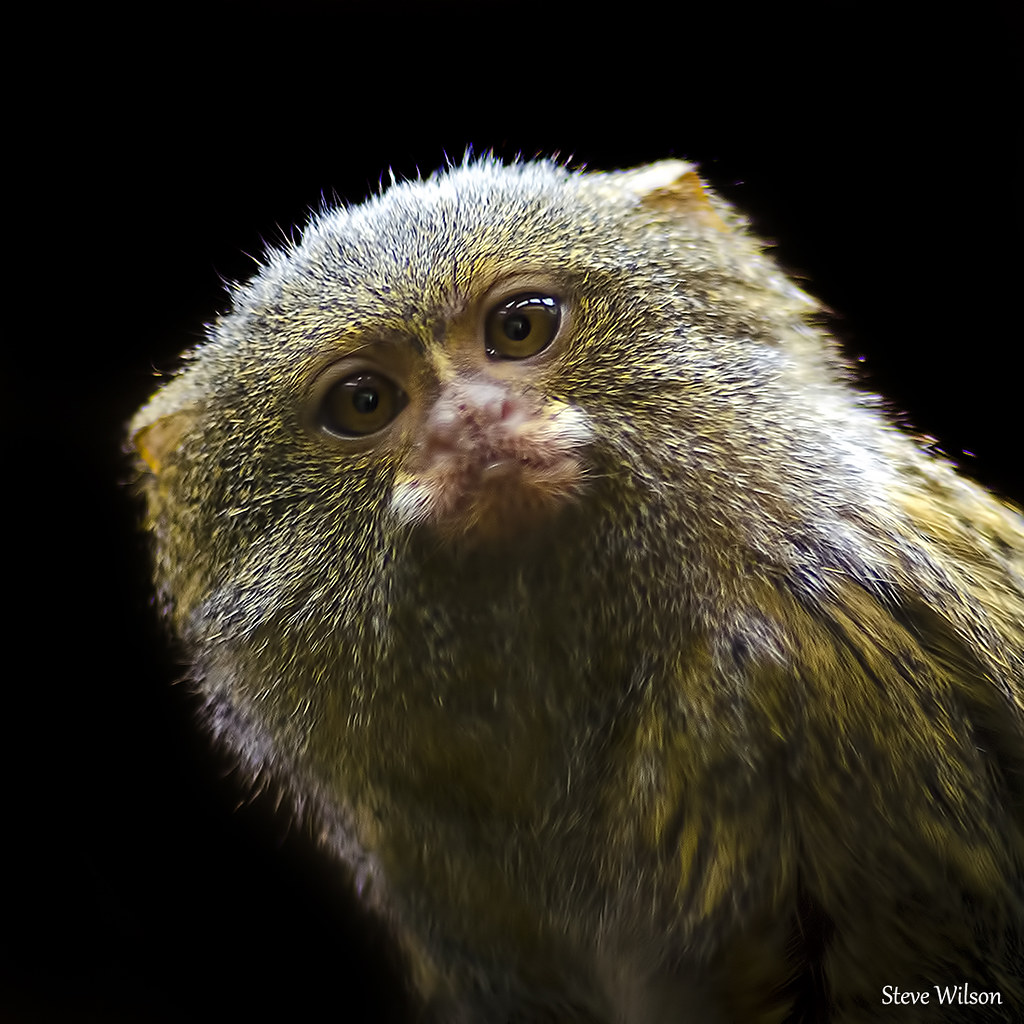This is a detailed and realistic close-up photograph of a monkey's face, captured by Steve Wilson, set against a stark black background that makes the subject stand out vividly. The monkey's fur exhibits a range of colors including tans, yellows, blacks, and greys, with hints of white around the face. Its eyes are a striking yellow, and it has a very light pink nose and mouth. The monkey is looking directly into the camera with an expressionless, almost inquisitive gaze. The superb detail of the photograph allows you to see individual strands of fur and pores on the monkey's nose, emphasizing its lifelike quality. The credit for the photo is subtly included in the lower right-hand corner.